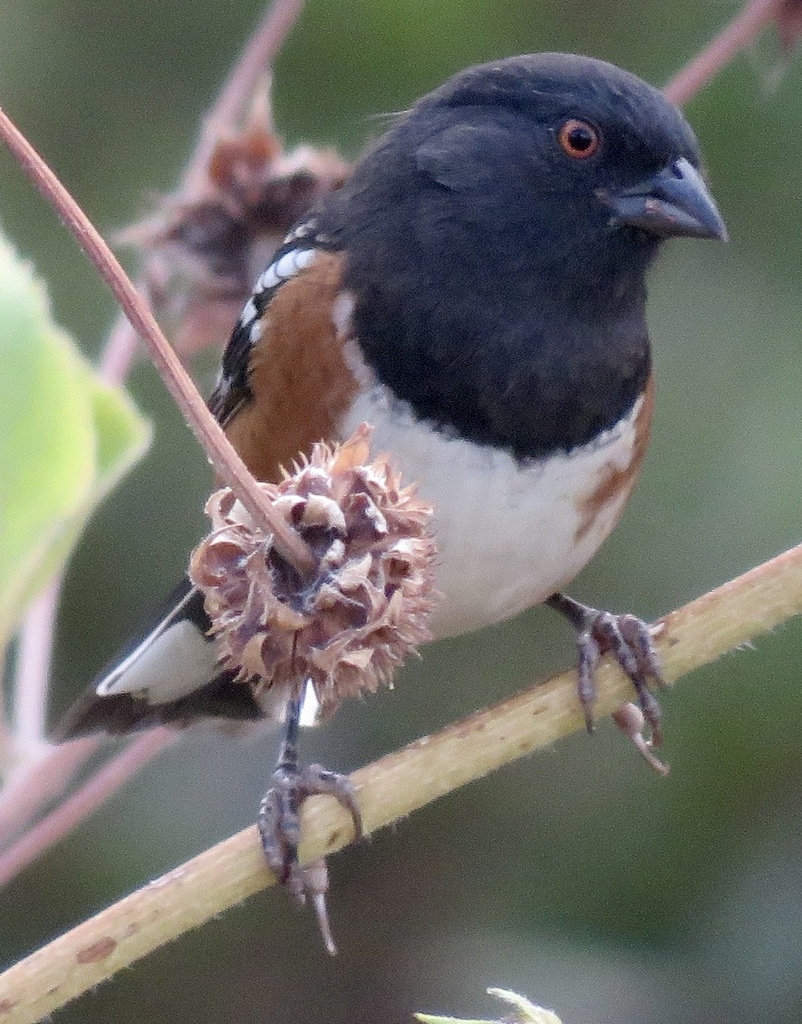In this detailed, zoomed-in image taken in nature, the main focus is a small bird, predominantly centered in the upper right portion of the frame, perched on a thin, light brown wooden stick that extends across the bottom of the screen. The background is blurred, with vibrant green leaves and some pink, prickly flowers adding depth and a natural setting. The bird itself is distinct with a striking black head, an orange eye with a black pupil, and a black beak. It has a white chest, brownish feathers on its sides and shoulders, and a back tip of the wing that is black and white. The bird's legs are dark brown, with grayish claws gripping the branch. No text is present in the image, allowing the viewer to focus purely on the natural beauty depicted.